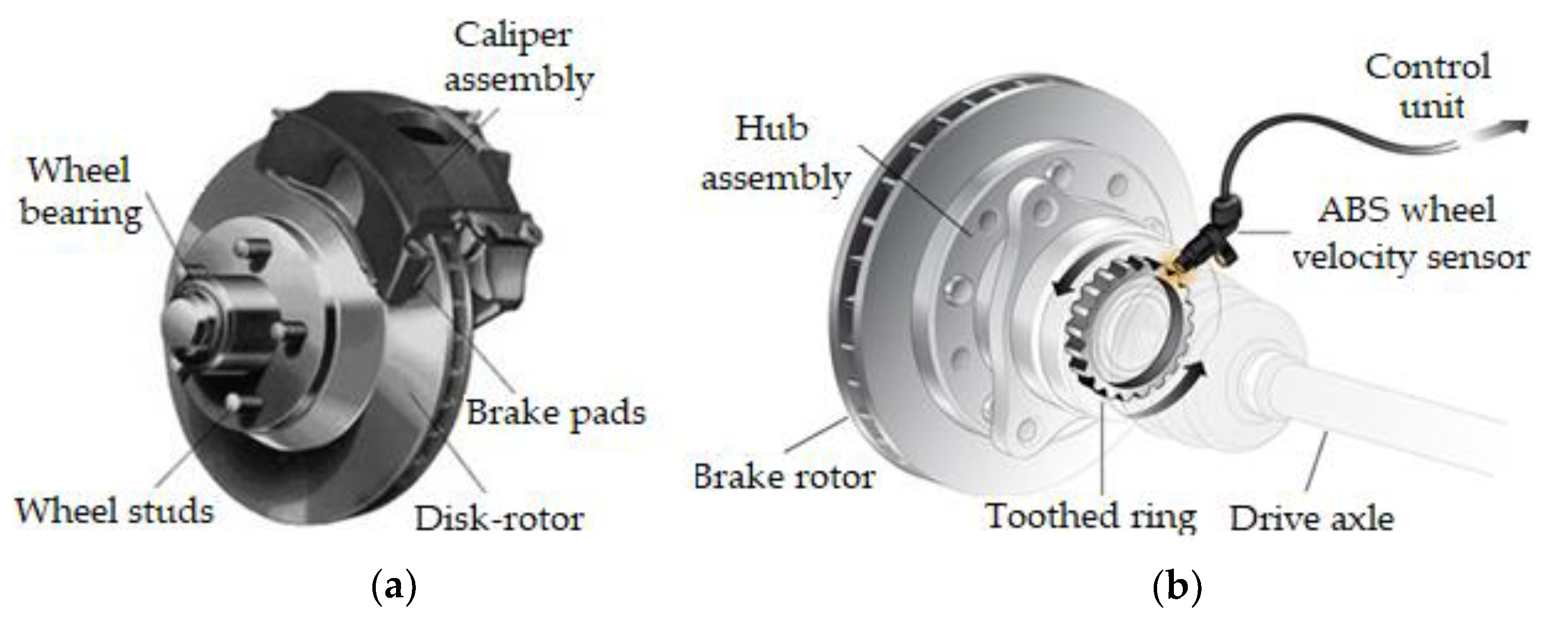This horizontal image vividly illustrates a deconstructed automobile braking system, split into two labeled sections: A on the left and B on the right, both adorned with detailed annotations. The left-hand side (A) showcases various metal parts in different shades of gray, with the caliper assembly standing out in a darker gray. Labels point to several components, including the disc rotor, brake pads, wheel studs, wheel bearing, and caliper assembly. The right-hand side (B) presents a partly transparent view to reveal its internal mechanisms, emphasizing the complexity of the system. Here, you see the hub assembly, brake rotor, toothed ring, drive axle, ABS wheel velocity sensor, and control unit, with notable features such as a tool with an attached wire. Both sides highlight the sophisticated, circular design of the braking system, essential for understanding the integral parts of automobile brakes.